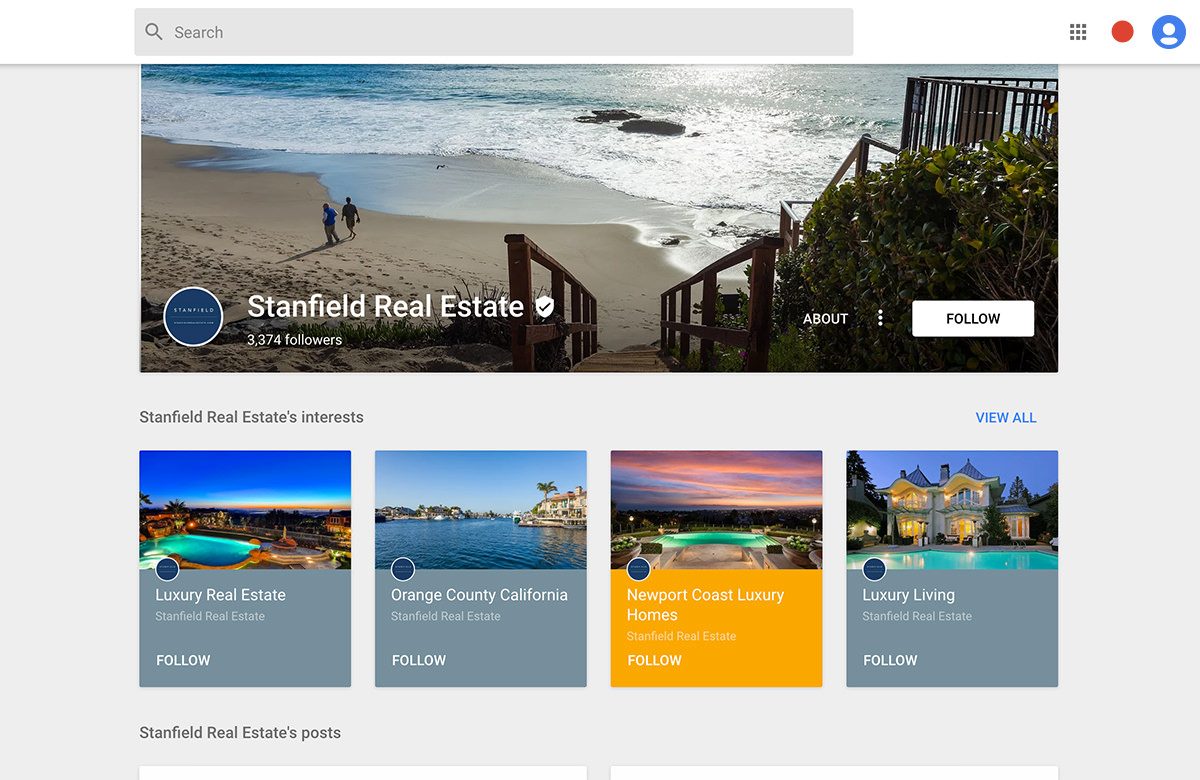Screenshot of a Minimalist Real Estate Website:

At the top of the webpage, there is a simple white navigation bar. Within this bar, a gray rectangle serves as the search field, bearing the placeholder text "Search" in gray font, accompanied by a gray magnifying glass icon on its left side. On the right end of the navigation bar, three distinct icons are visible: an array of nine gray dots arranged in three rows of three, a red circle, and a blue circle featuring the white silhouette of a person.

Below the navigation bar, the main content area of the page has a light gray background. Dominating the top portion of the content is a panoramic photograph of a beach with brown sand. In this serene image, two distant figures walk hand-in-hand along the shoreline where the waves gently break, casting visible shadows under the bright sunshine. The scene evokes a sense of tranquility and connection.

In the lower left corner of the photograph, the text "Stanfield Real Estate" is displayed alongside a verified check mark, indicating authenticity. Just below this, the follower count stands at "3,374 followers." In the lower right corner, white text reads "About," beside which is a "Follow" button.

Further down the page, a heading declares "Stanfield Real Estate's interests," followed by a series of images showcasing luxurious mansions and other properties, giving viewers a glimpse into the high-end real estate offerings available through Stanfield Real Estate.